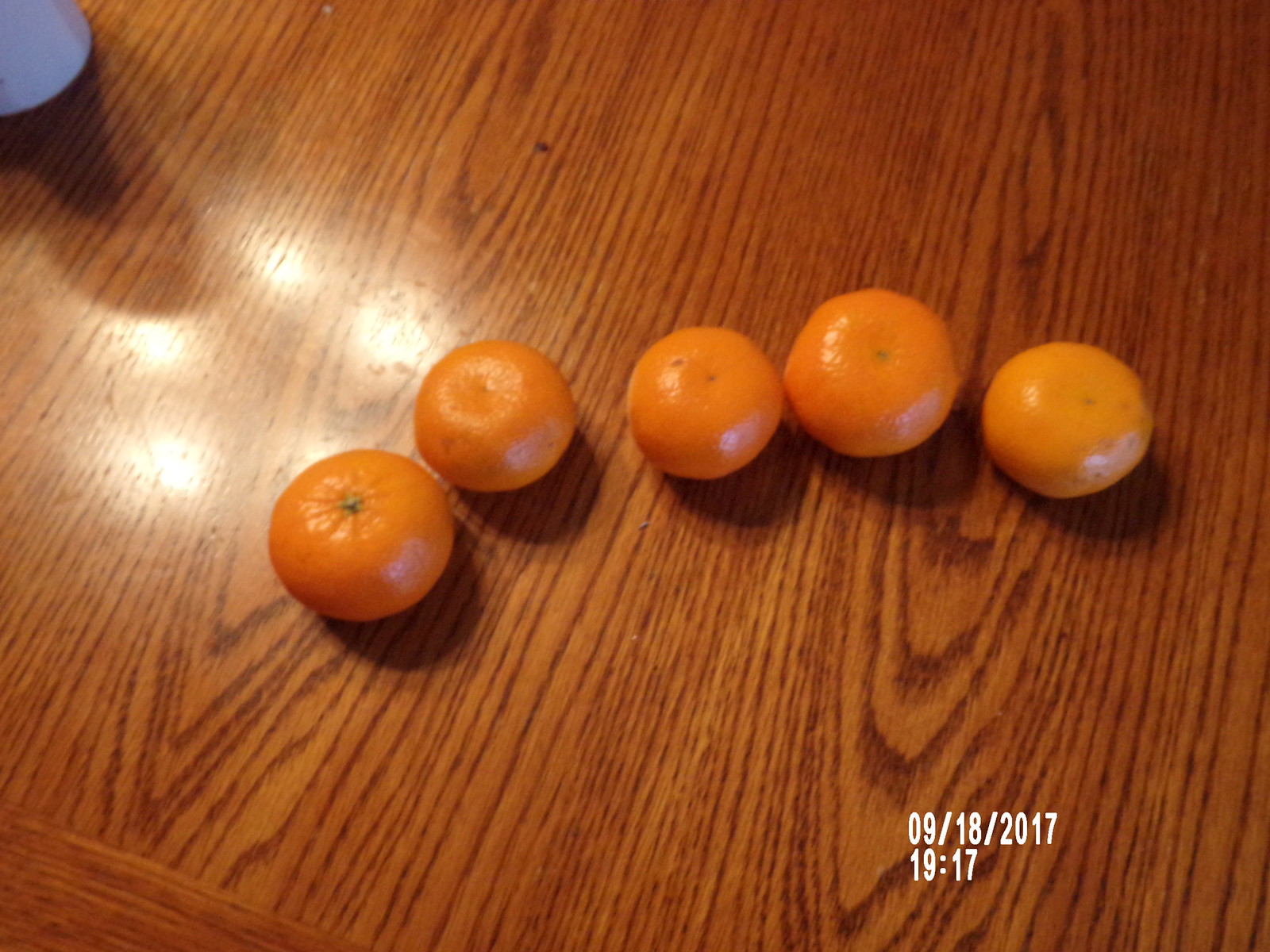This image showcases five small tangerines arranged in a curved line on a brown oak grain wooden tabletop. The tangerines, approximately a couple of inches in diameter, display a waxy sheen, suggesting they might have been polished before packaging. While most of the tangerines sit with their stems facing down, one is positioned stem side up. Overhead lighting creates a ring of reflections on each tangerine, giving the bottom right side of each fruit a lighter appearance. In the upper left corner, the base of a white ceramic mug or container casts a shadow on the table. The photograph bears a watermark in the bottom right corner, displaying the date "09-18-2017" and the time "1917," pinpointing when the photo was captured.